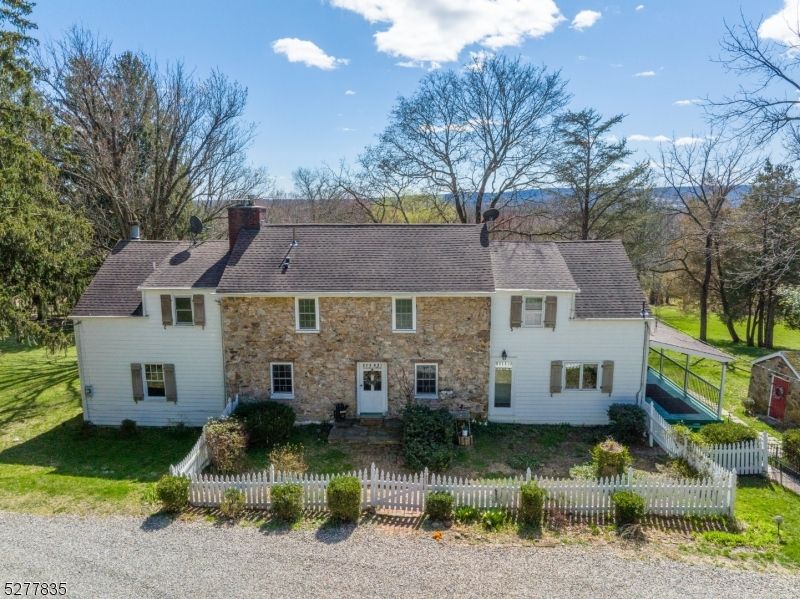This aerial image showcases a sprawling, two-story house set in a remote, picturesque countryside, surrounded by lush green landscapes and a striking backdrop of valleys and tall, leafless trees. The central structure of the home is constructed from light beige bricks, giving it a solid and traditional appearance. The house features numerous traditional-style windows with brown trims and storm covers in light wood color, enhancing its rustic charm.

The home has two prominent extensions on either side, both painted white with vinyl siding. The left and right extensions appear to be more recent additions, seamlessly integrated into the original structure. The roof is robust and brown, complementing the overall aesthetic of the residence.

The property is enclosed by a quaint white picket fence, encircling a well-maintained green yard adorned with various bushes and green plants. Just behind the main entrance, there's a serene white picketed backyard. A small storage shed with a red door is situated to the right of the house, adding to the practicality of the estate.

In front of the house, a large driveway extends into the expansive property. The background reveals a breathtaking mountainscape beneath a bright blue sky dotted with fluffy white clouds, contributing to the image's vibrant and serene ambiance.